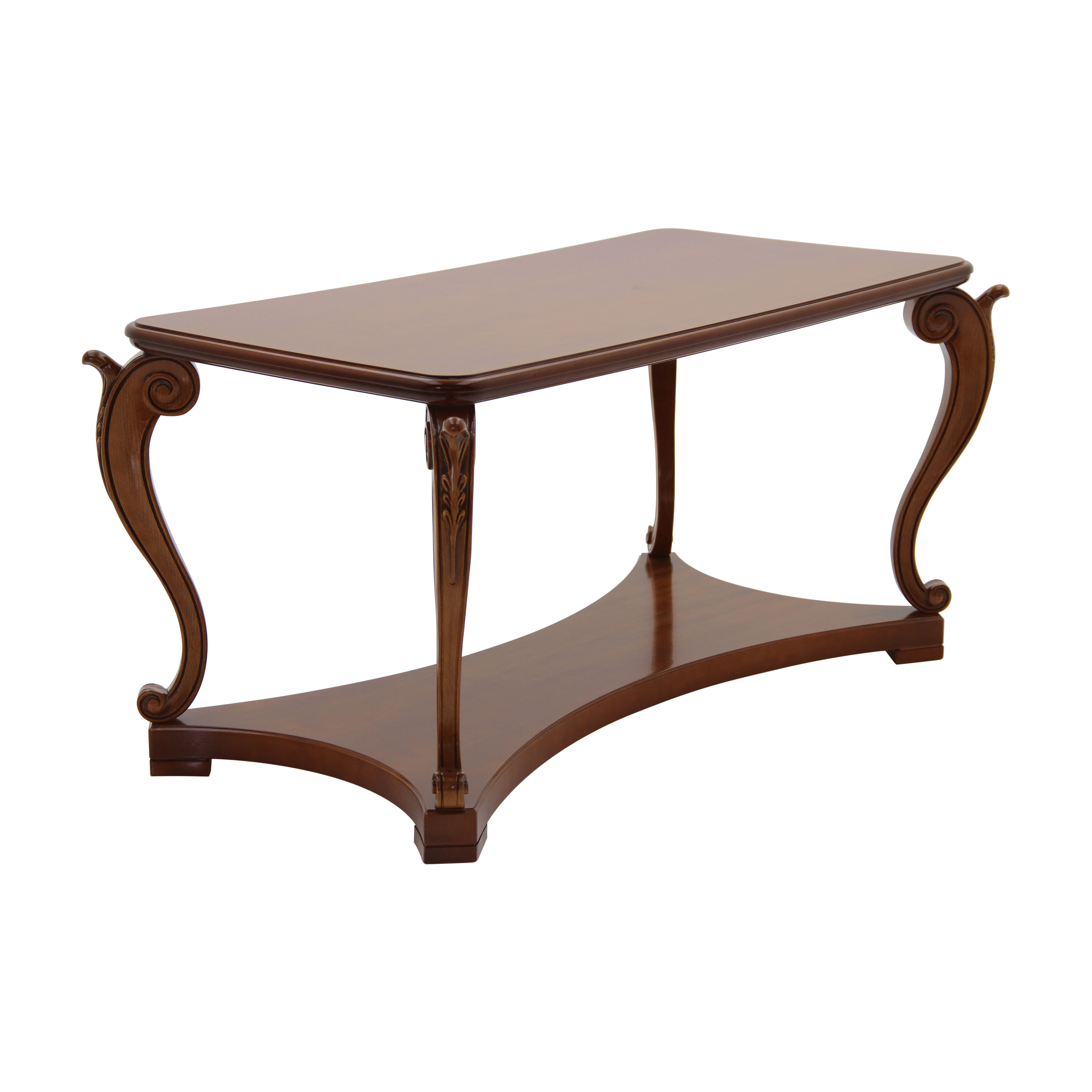This professionally photographed image showcases an ornate wooden table set against a pristine white background, highlighting its finely crafted details without any distractions or shadows. The table features a rectangular flat top and a lower curved shelf, supported by four intricately designed legs. These legs resemble undulating 'S' shapes, with decorative carvings reminiscent of fish, complete with large circles at the top and smaller circles at the base. The bottom panel, also curved inward, complements the overall elegant design. The table's sophisticated appearance suggests it is a high-quality, substantial piece, ideally suited for a living room setting, perhaps for holding newspapers or as an accent piece in front of a couch or TV.